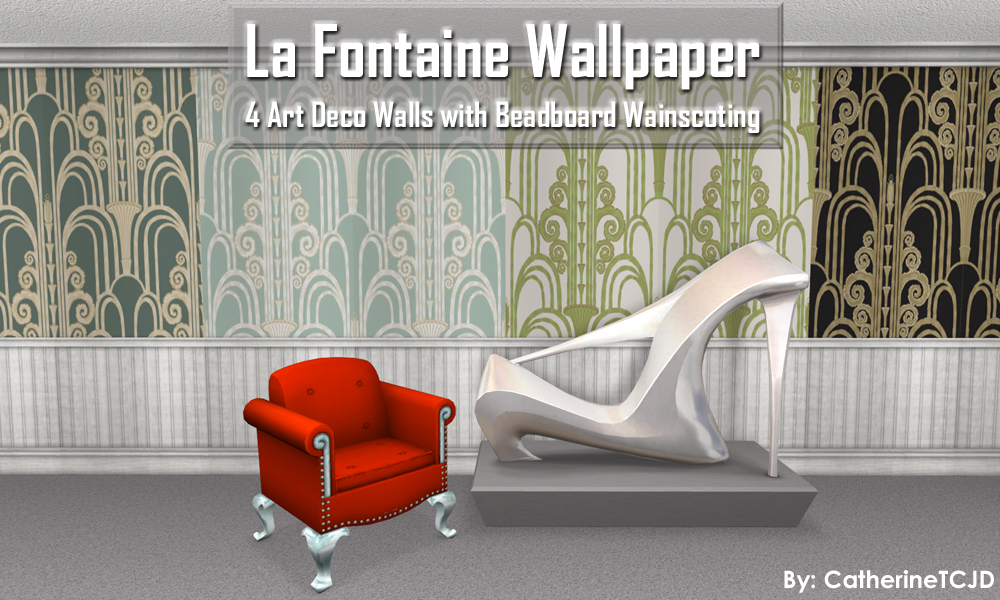The image is a digitally-designed advertisement featuring "La Fontaine Wallpaper" as declared in white block lettering at the top. Below this heading, smaller text reads, "For Art Deco walls with beadboard wainscoting." The background showcases four variations of Art Deco wallpaper, each exhibiting the same intricate design but in different color schemes: a jet-black background with gold lining, a white background with green lining, a pale green background with white lines, and a mid-to-dark green background with white lines. These wallpapers are reminiscent of the towering, loopy swirls reminiscent of the Empire State Building's aesthetic. 

The lower third of the image reveals a grey, carpeted floor with beadboard wainscoting in a pearlescent white finish. The central focus is a bright red armchair with silver accents and legs, positioned next to a piece of art that resembles a large, abstract stiletto heel. The armchair and art piece appear to be computer-rendered. In the bottom right corner, in white text, it reads, "By Catherine T.C.J.D."